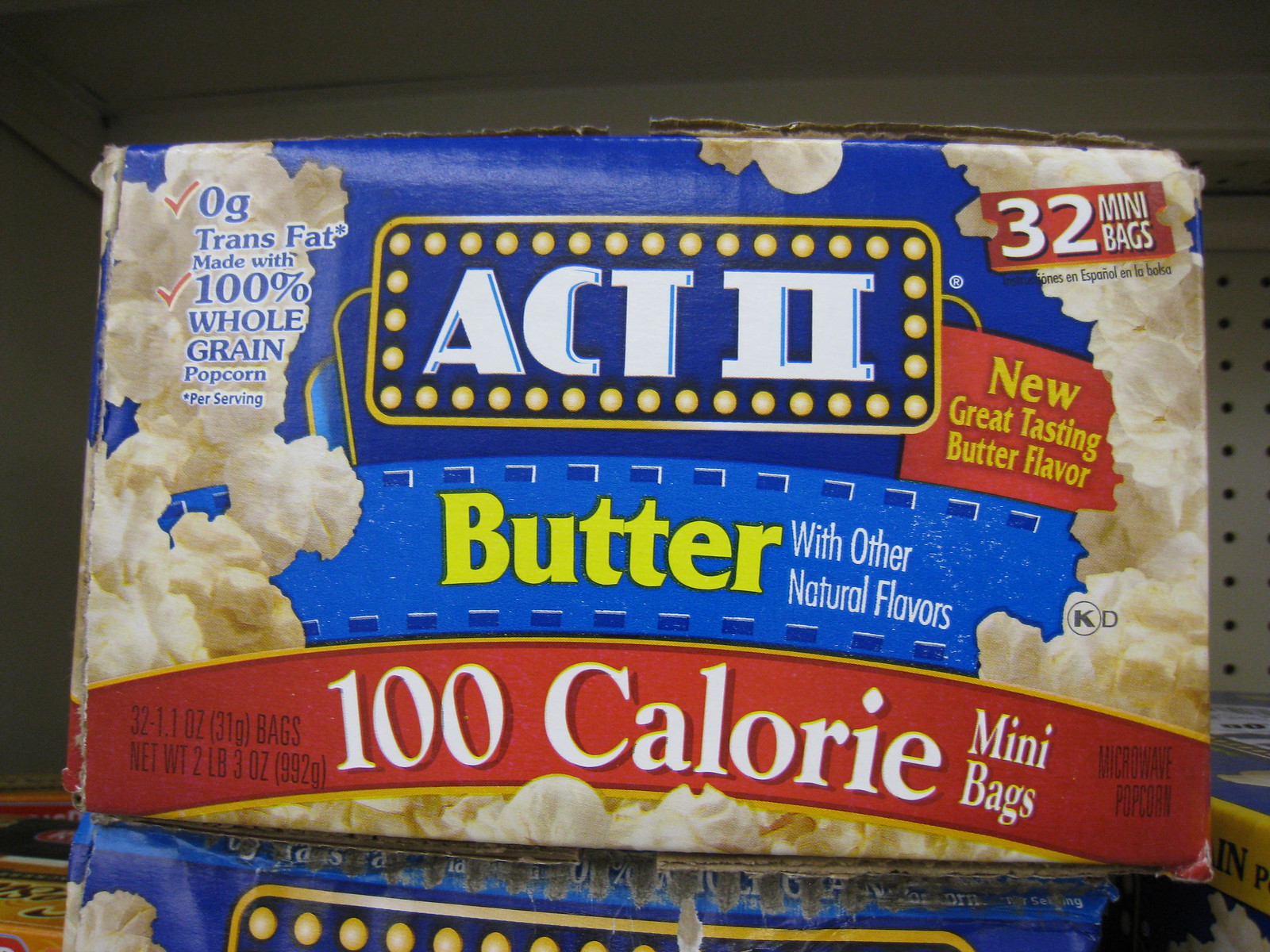The image shows a close-up photograph of an old, slightly battered box of Act 2 popcorn, which is likely positioned on a supermarket shelf. The horizontally rectangular box features a vibrant indigo blue background, adorned with images of popcorn cascading down the left and right sides and across the bottom. Prominently displayed at the top is the brand name, "Act 2," written in white lettering with a yellow rounded rectangle border decorated with small yellow globes. Underneath this, a banner resembling a movie reel announces "Butter" in yellow letters, accompanied by the phrase "with other natural flavors" in white. A red banner below that indicates "100 calorie mini bags." On the top right corner of the box, a red movie ticket-shaped graphic states "32 mini bags." Additional details on the left-hand side of the box include "Zero Grams" and "Made with 100% whole grain popcorn per serving" in blue writing among the popcorn kernels.